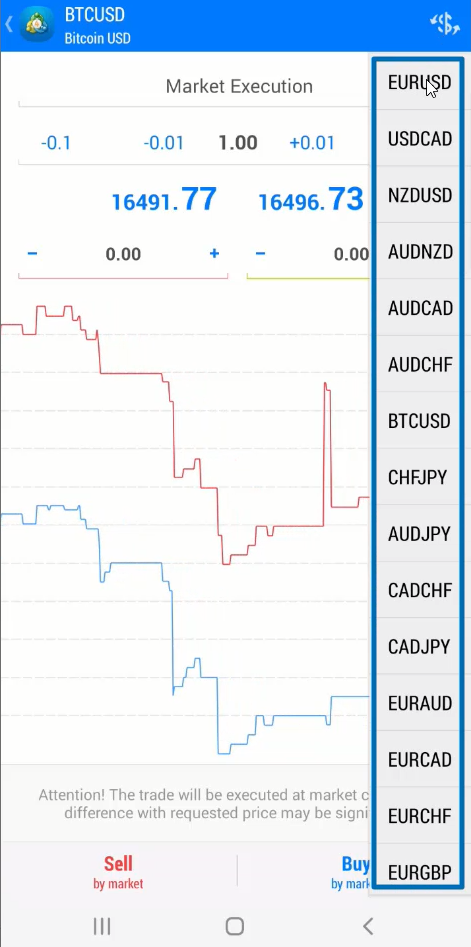This screenshot captures the interface of a cryptocurrency conversion app on an Android smartphone. At the top left, it displays "BTC USD," indicating the conversion from Bitcoin to USD. Beneath this, you can see "Bitcoin USD" paired with a small Bitcoin emblem for visual clarity. On the far right, there is a dollar sign emblem with two arrows pointing up and down, symbolizing the swap function.

Directly below the top section, the app features a list of various currency conversions beyond Bitcoin to USD. These include:

- EUR to USD
- USD to CAD
- NZD to USD
- AUD to NZD
- AUD to CAD
- AUD to CHF
- BTC to USD
- CHF to JPY
- AUD to JPY
- EUR to AUD
- EUR to CAD
- EUR to CHF
- EUR to GBP

In the center of the screen, a graph visually represents the fluctuations in Bitcoin's value over time. As per the current data displayed, the value of Bitcoin stands at approximately $16,500.